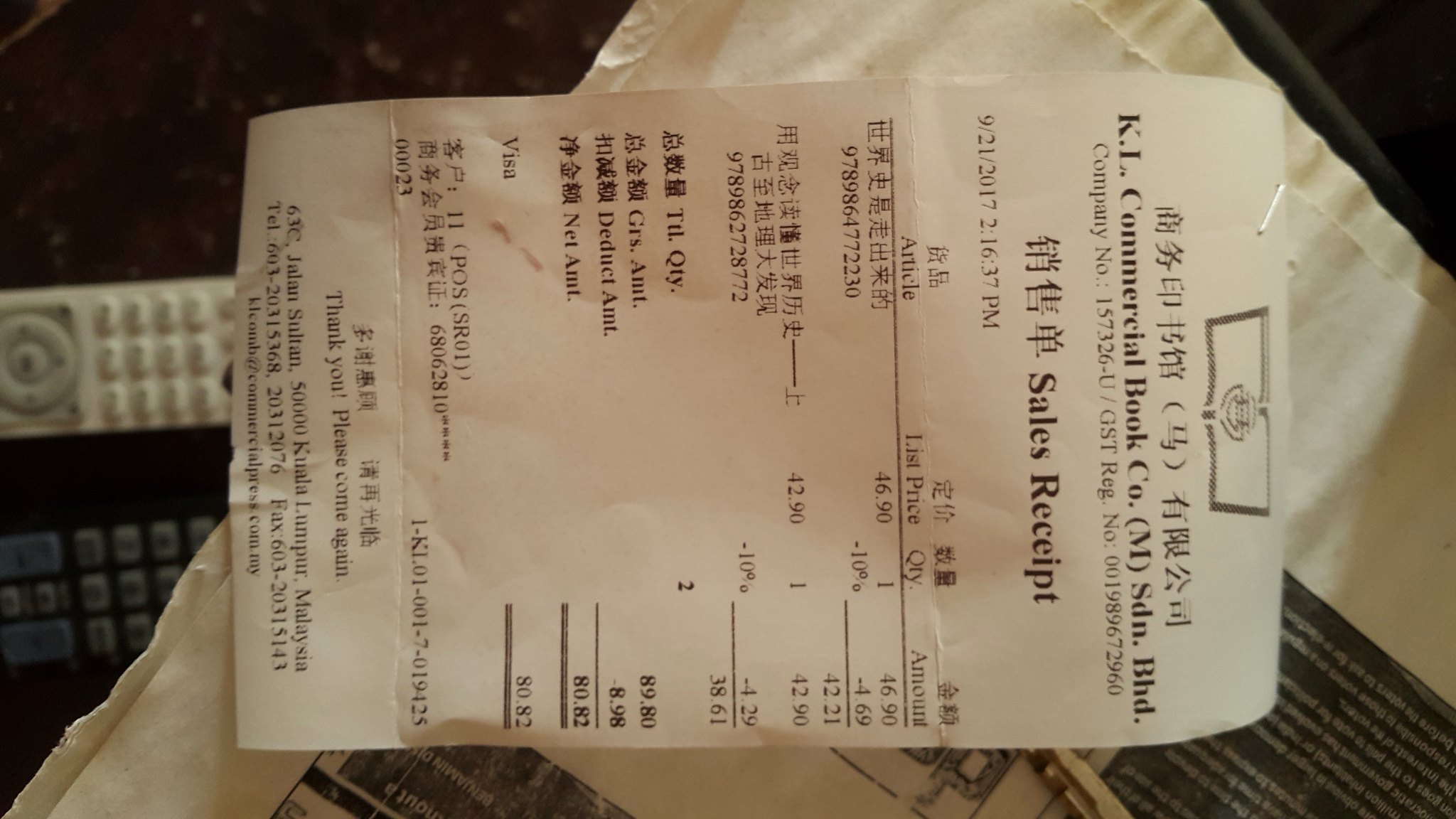This image depicts a sideways-receipt from R.I. Commercial Book Company, located on MSDN Boulevard. The top of the receipt is oriented towards the right side of the photo. The header features both Chinese or Japanese characters alongside English text. Beneath the company’s name and address, there is a company identification number, followed by the terms "Sales Receipt" presented in both the Asian language and English. The receipt details a total purchase amount of $89.80. Following a deduction of $8.98, the final amount comes to $80.82. The bottom of the receipt politely thanks the customer with a "Thank you, please come again" message. The specific items purchased are not listed in the photo.